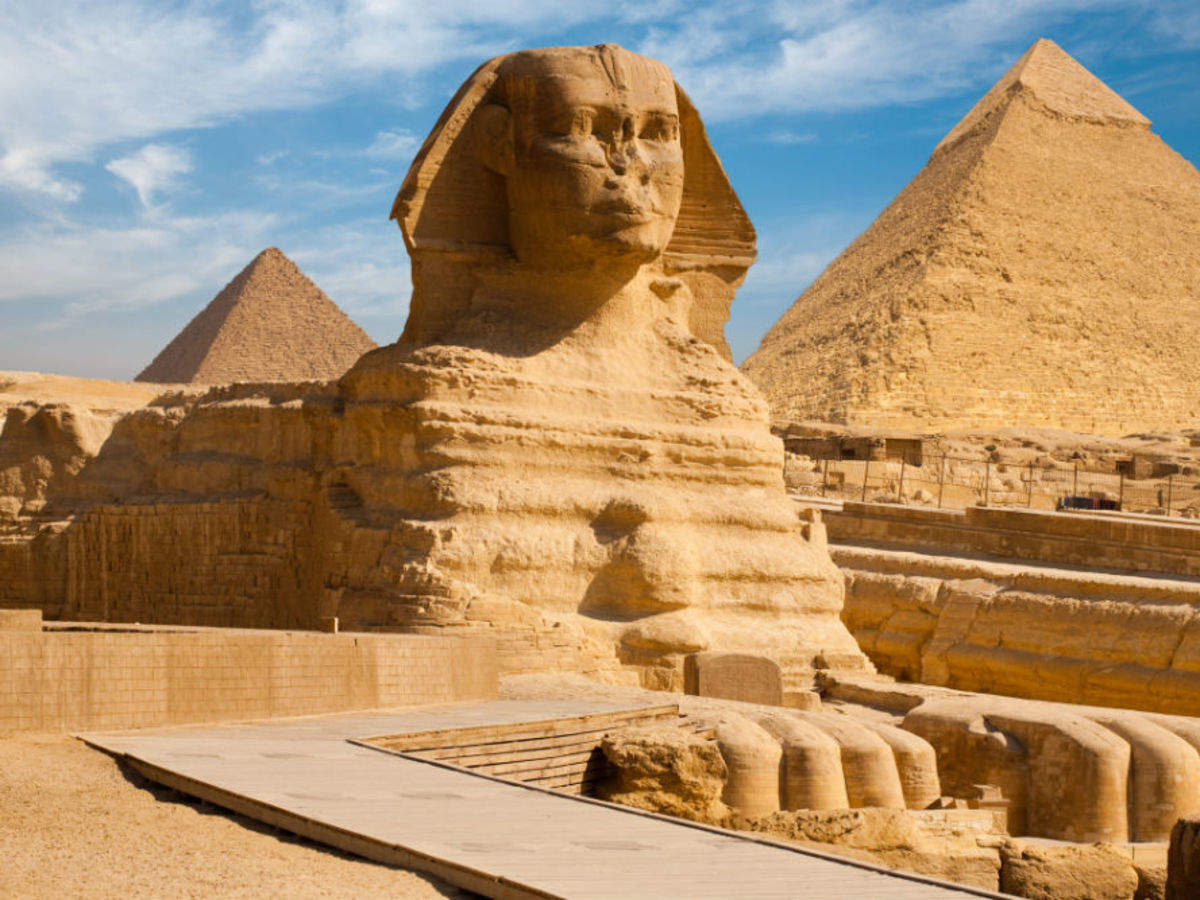This photograph captures the iconic Sphinx at Giza positioned centrally, set against a backdrop of two pyramids under a clear blue sky. The Sphinx, an Egyptian monument featuring a human head adorned with a headdress and a lion's body, lies with its paws extended forward. Noticeably, the Sphinx's nose is missing, and its intricate details show varying shades of brown and yellow. An L-shaped walkway leads up towards the Sphinx, curving to the right, drawing the viewer's eye to the majestic statue. To the right in the background stands the Great Pyramid, characterized by a more intact peak and a weathered, chunky lower section. The pyramid on the left, farther in the distance, appears entirely worn, with a rough, uneven surface, contrasting with the more preserved state of the Great Pyramid.